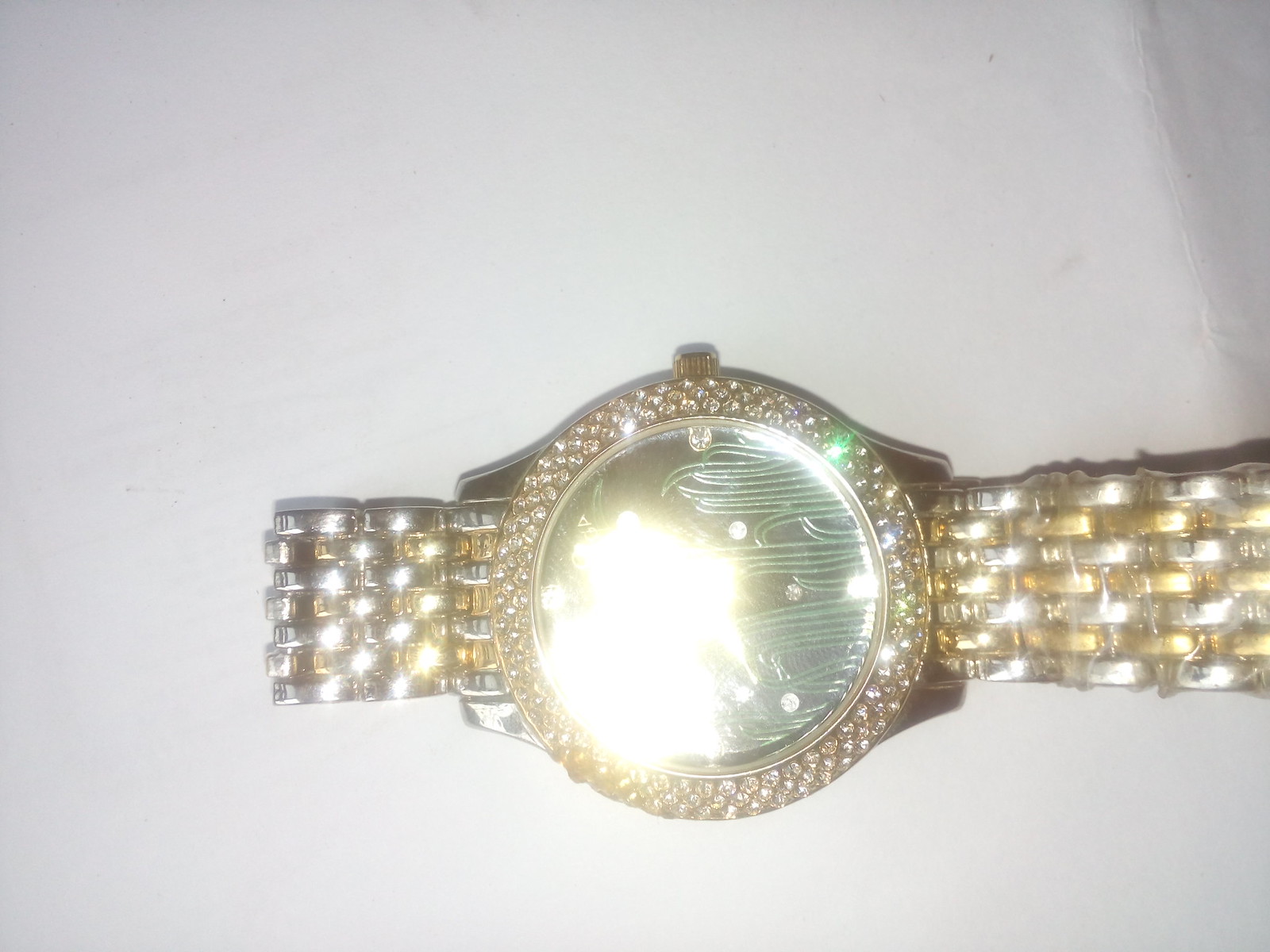The photograph showcases a luxurious wristwatch positioned off-center towards the bottom right against a clean white or gray background. The watch itself is composed of shiny metallic elements, predominantly gold, with intricate, metallic striped patterns on the band. The circular face of the watch is highly reflective, casting bright white light that obscures the numbers or the time, and it seems to feature faint green lines reminiscent of an artistic grass motif. Encircling the watch face are numerous small, sparkling stones that resemble diamonds, further enhancing its opulent appearance. Despite the bright reflections and potential scratches on the glass, the overall impression is one of an elegant, possibly expensive accessory, though the absence of clear text or discernible time makes it challenging to verify its authenticity.